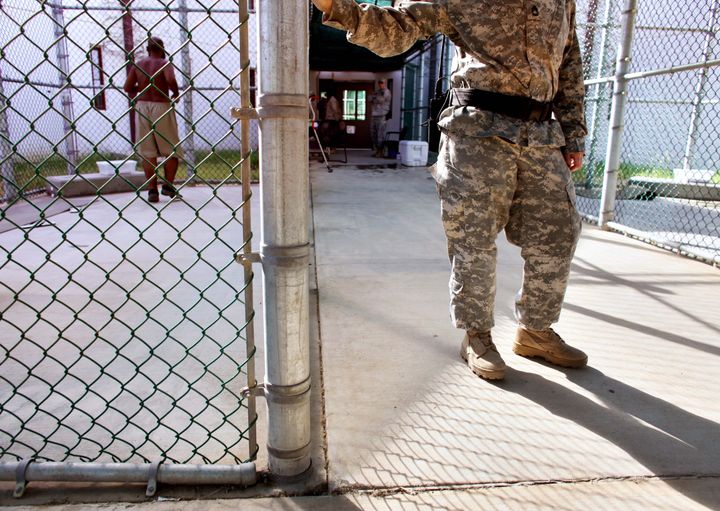The photograph depicts a realistic, horizontally-oriented scene centered around a concrete-floored, daytime outdoor area enclosed by a chain-link fence. In the foreground, a soldier dressed in olive beige camouflage and beige boots, with a visible black belt, stands guard, holding a metal post that is part of the fenced enclosure. The soldier is shown from the shoulders down. Inside the fenced area to the back left, an African-American man, shirtless and in beige pants, is walking away from the camera. Further back into the facility, a hallway extends into the distance, where two additional figures in similar military uniforms are barely discernible. The entire setting suggests a restricted or secure facility, such as a prison or military holding area. A window at the far rear of the hallway can be faintly seen, giving a glimpse into the interior of the facility. The image lacks any text elements and maintains a straight-forward, documentary style without any intentional artistic composition.